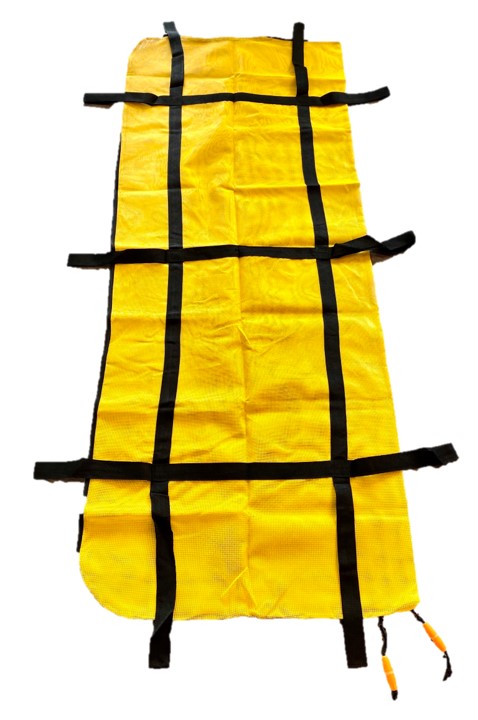This image showcases a bright yellow, almost banana-colored cloth material laid against a stark white background. The item appears to be a fabric, possibly nylon or flannel, and possesses a rectangular shape with noticeable creases that suggest it has been previously folded. Prominent black nylon straps constitute a crisscross pattern over the yellow surface, arranged with three horizontal straps and two vertical ones, evoking a checkerboard-like design. These straps could function as compression mechanisms, potentially suggesting a use in wrapping or securing objects. The bottom right corner of the item features two black drawstrings or toggle cords, each adorned with yellow beads, which might serve for tightening or closure purposes. Along the left-hand side, beginning from the bottom, a black zipper is visible but it does not extend to the full length of the item. The exact purpose of this object is unclear—it could range from a storage bag or carrying case, possibly for camping equipment or large items, to a safety device like an inflatable raft or evacuation sheet.